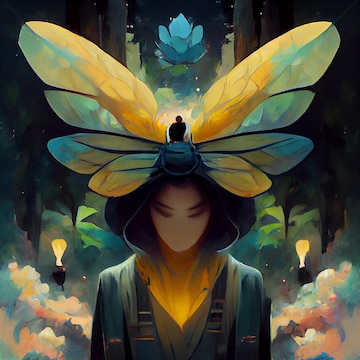In this vibrant, digital artwork reminiscent of anime or pop art, the central figure is a person wearing a hooded yellow turtleneck. Their face is mostly blank, save for two black slashes representing eyes. The figure stands with their head slightly bowed, and a large, yellow butterfly or butterfly wings appear to emerge from the top of their head. This striking imagery is set against a backdrop of abstract, blurred shapes in dark gray or light black tones. A lighter blue lotus flower, transitioning to a darker blue at the base, floats above their head. The background evokes a forest-like scene with hues of green suggesting trees and foliage. Puffy, medium-yellow or light-orange clouds hover around, while two yellow light bulbs flank the figure on the left and right. The scene conveys a blend of natural elements and surreal, fantastical features, creating a captivating and mysterious atmosphere.